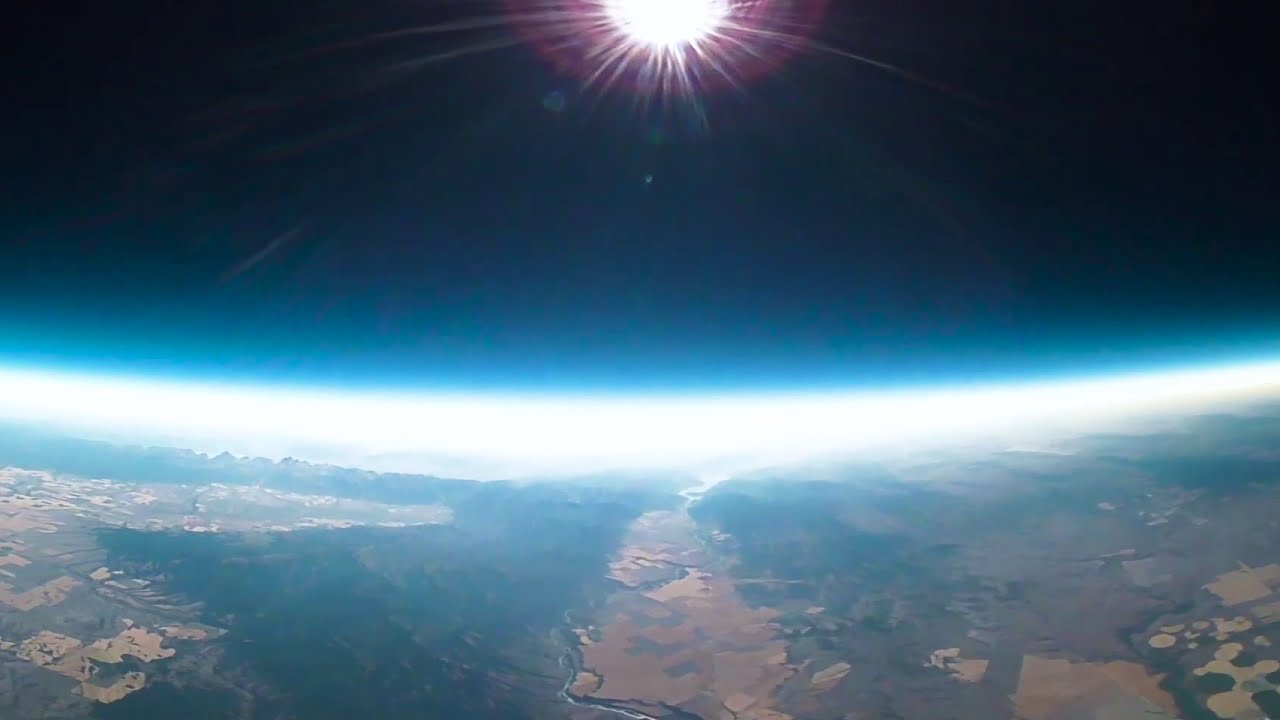This captivating photograph appears to have been taken from a high-altitude vantage point, likely from a spaceship in outer space. The image is rectangular and oriented horizontally. At the very top of the picture, a brilliant white light is visible, likely the sun or a bright star, casting rays in all directions. Surrounding this white ball of light is a soft halo effect with gentle hues of purple and red semicircles.

Beneath the sun is the vast expanse of outer space, appearing as a deep, dark black horizontal band stretching across the image. Below this darkness, the view transitions into a glowing blue horizontal stripe, which may represent the Earth's atmosphere. Immediately below this blue is a thin white stripe, indicative of atmospheric layers or clouds.

The lower half of the image is dominated by the Earth, which showcases its natural beauty. You can see sprawling blue oceans and vast landscapes. The land appears in various shades of brown, with some areas looking rocky or muddy, along with patches of green that suggest forested or vegetated regions. The central area seems to feature a river or brown water body, flanked by lighter and darker brown fields, perhaps agricultural land. In the background on the left side, faint outlines of buildings suggest a city or town. Overall, the photo captures the grand scale and diversity of Earth's surface from an awe-inspiring perspective in space.